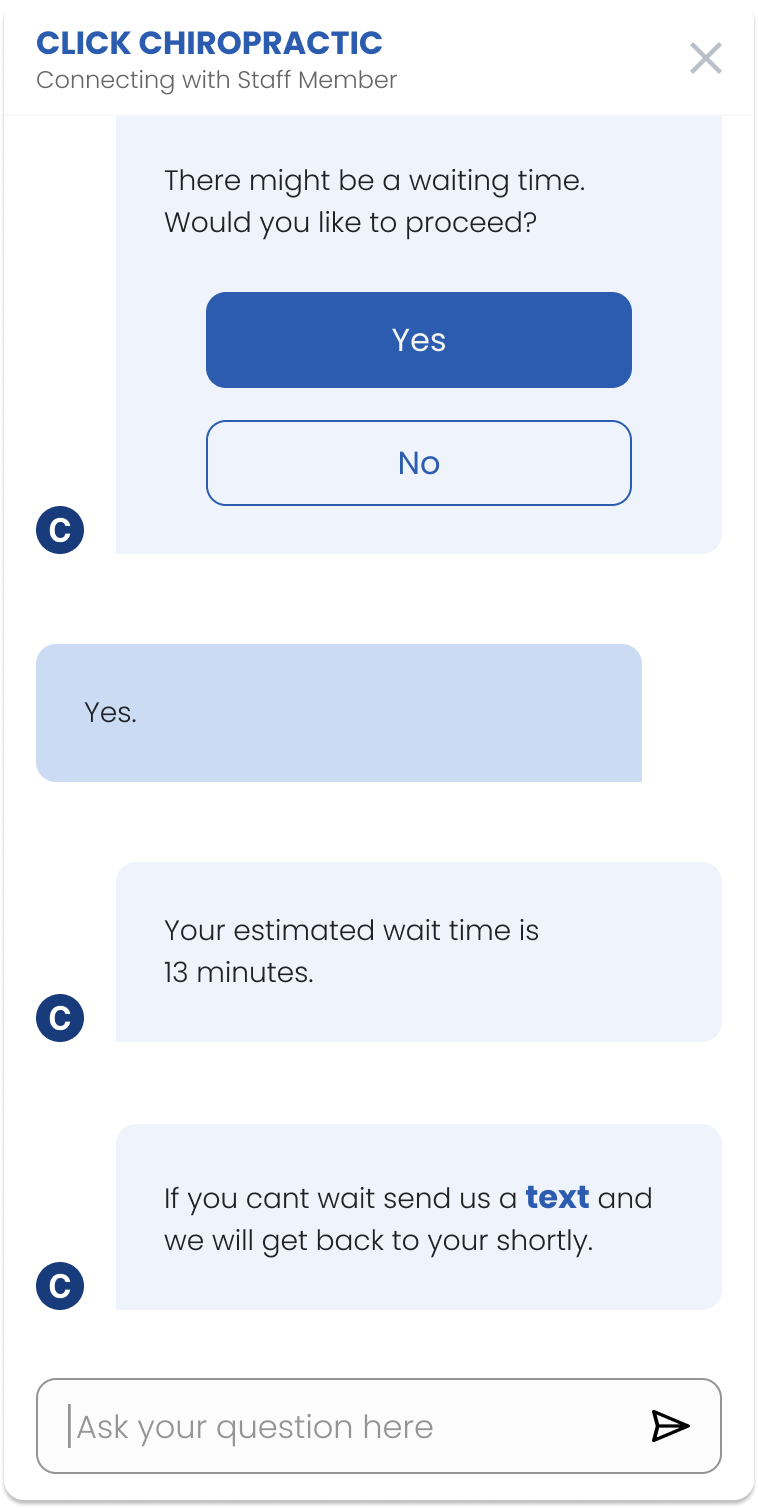The image depicts an interface of a chat application used for consulting a chiropractic service. At the top of the interface, there is a blue banner with text. On the top left corner, the banner reads "Click Chiropractic" while in the top right corner, there is an 'X' button for closing the chat. Just below the blue banner, in gray text, it says "Connecting with Stephanie."

A prominent light blue box at the top of the chat window informs the user that "there might be a waiting time." Below this notification, there are two buttons: a solid blue button labeled "Yes" and a blue-outlined button labeled "No." The user selects "Yes," leading to a light blue speech bubble that acknowledges the choice with a smile. After waiting for 30 minutes, the chatbot sends another message saying, "If you can't wait, text, and we will get back to you shortly. Thank you."